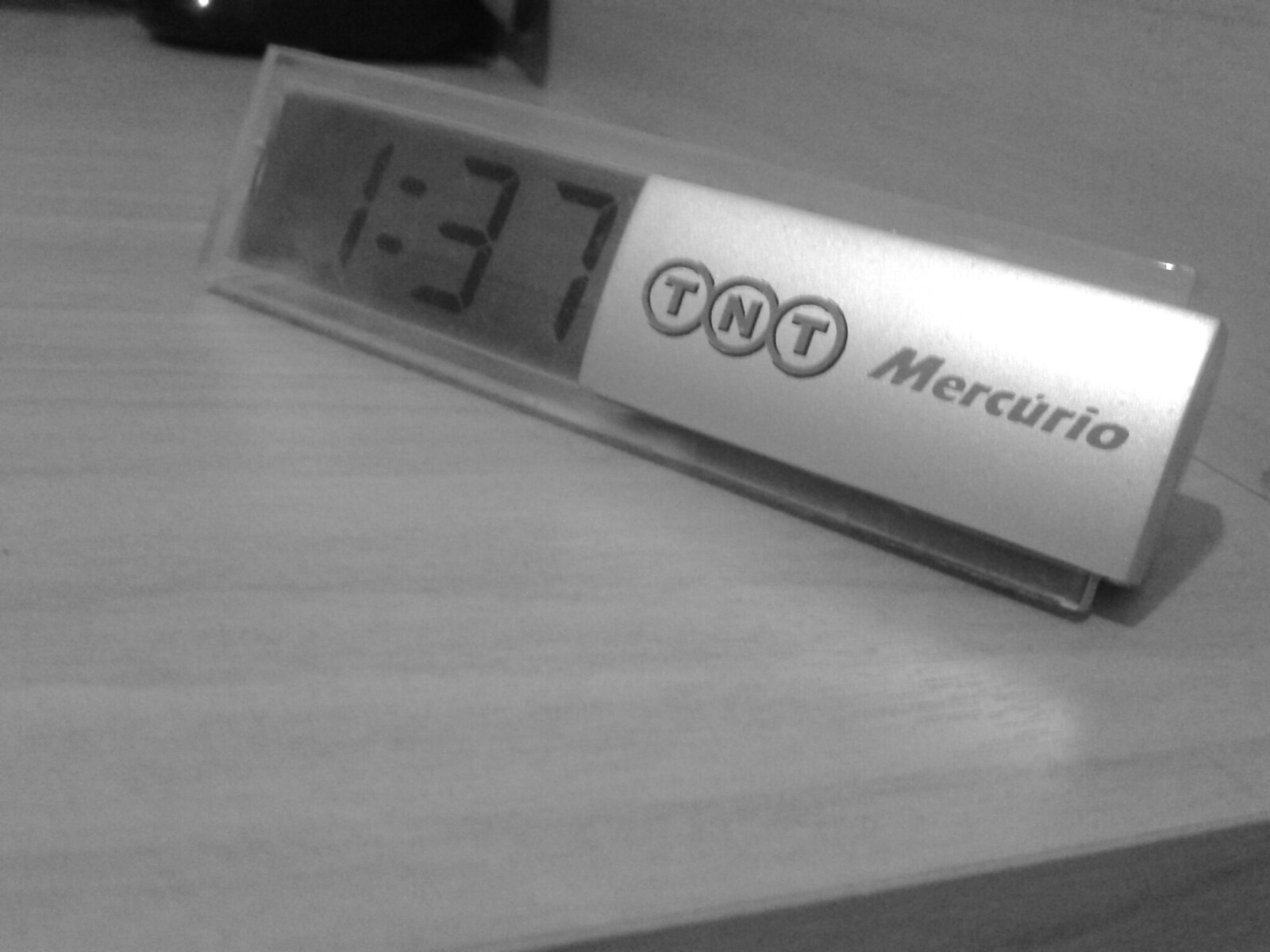This is a detailed black-and-white photograph showcasing a long, narrow, rectangular digital clock resting on a wood-grained tabletop, likely a desk or dresser. The clock displays the time as 1:37 with black digital numbers set against a dark gray face. To the right of the display, the clock features a shiny silver section with the TV network logo "TNT"—each letter encased in a gray circle. Further along, it displays the word "Mercurio" in block letters. The clock has clear plastic borders, adding to its sleek design. In the upper left corner of the image, there's a small black object lying on the table, adding a subtle element of detail to the composition.